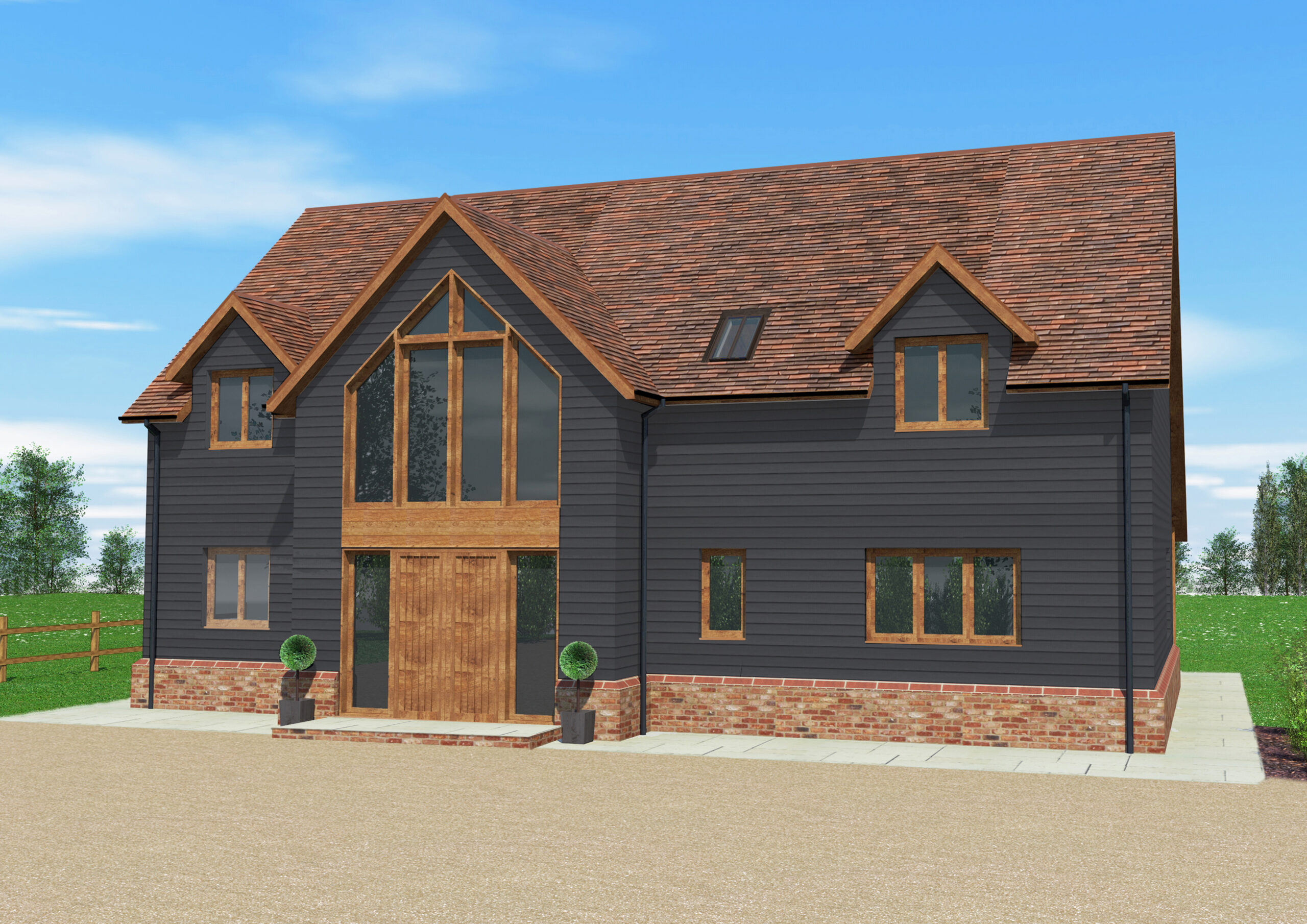This image is a detailed, digital 3D illustration of a one-story house with an attic, likely created for an architectural presentation or sales pitch. The house has a dark grey exterior made of wooden slats, complemented by a trim of red brick at the foundation. The roof is covered with wooden tiles. Prominently, the front features a large window and a main entrance that appears quite tall, with brown wooden doors flanked by perfectly round green bushes in grey planter boxes. There are also dormer windows positioned on either side of the entrance. The house sits on a brown gravel driveway, and the surrounding environment includes green fields, a brown fence, and some distant trees under a blue sky with white clouds. The overall aesthetic blends modern and country-barn styles.